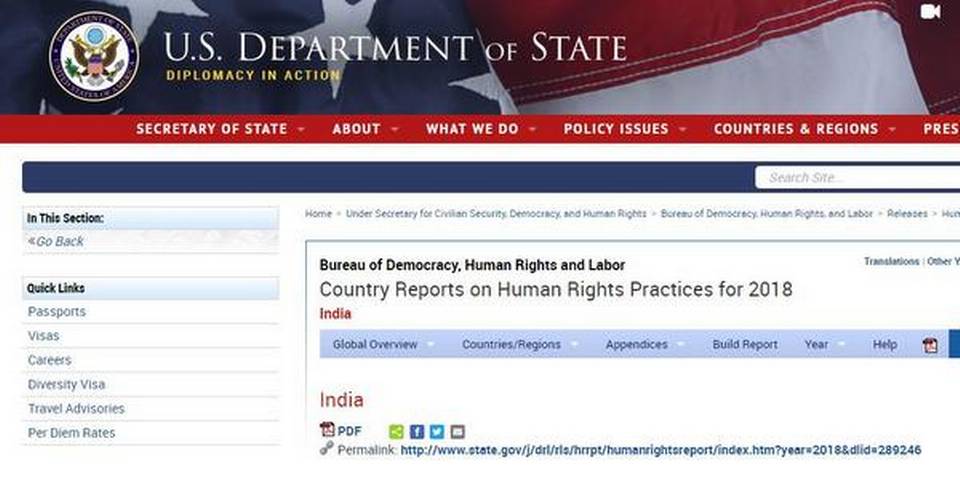The webpage from the US Department of State prominently features the header "US Department of State: Diplomacy in Action" on a background. An American flag image underscores the patriotic theme, and to the left, a round, blue Department of State watermark adorned with an eagle signifies authenticity.

In the top right corner, a video camera icon hints at available multimedia content, labeled "Secretary of State." The main navigation bar includes dropdown headers: Secretary of State, About, What We Do, Policy Issues, Countries, and Regions, followed by a partially visible "Press" section—each dropdown presented in light red against a red bar, with text in white.

Beneath the navigation, a blue rectangle houses a search bar labeled "Search Site." The breadcrumb trail shows the user's navigation pathway: Home > Undersecretary for Civilian Security, Democracy, and Human Rights > Bureau of Democracy, Human Rights, and Labor > Releases. 

In another prominent rectangle, the title "Bureau of Democracy, Human Rights, and Labor Country Reports on Human Rights Practices for 2018 – India" appears. Below it, a light blue menu offers further navigation options: Global Overview, Countries/Regions, Appendices, Build Report, Years, Help, culminating with a PDF icon on the far right.

The country name "India" is highlighted in red beside the PDF icon, accompanied by various social media icons. A permalink is provided for direct webpage access: [US Department of State Human Rights Report](http://www.state.gov/J/DRL/RLS/HRRPT/HumanRightsReport/index.htm?year=2018&DTLID=289246).

To the left, two smaller sections appear: "In This Section" with an arrow pointing back and a "Quick Links" list including Passports, Visas, Careers, Diversity Visa, Travel Advisories, and Per Diem Rates.